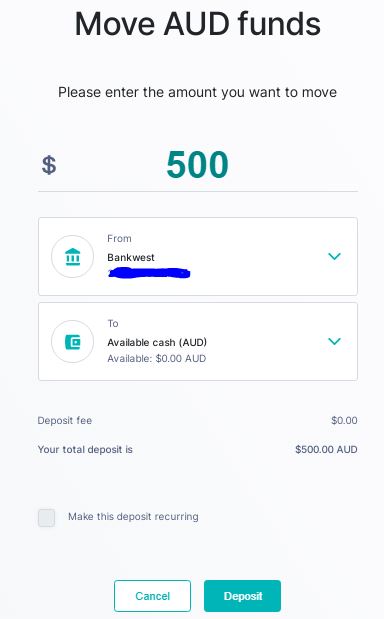The image shows a screenshot of a bank's online funds transfer page with a light gray background. At the top in bold black text, it reads "Move AUD Funds." Just below, there are instructions in smaller typeface saying, "Please enter the amount you want to move." An input line with a dollar symbol indicates an amount of 500 AUD is entered.

Beneath the input line are two rectangular selection boxes labeled "From" and "To." The "From" box shows "Bank West" with a corresponding logo and a dropdown arrow. The "To" box shows another bank logo with a label indicating "Available Cash: $0.00 AUD," and it also has a dropdown arrow.

At the bottom of the page, it states the deposit fee as $0.00 AUD, and the total deposit amount is confirmed as 500 AUD. A checkbox option is available for making the deposit recurring. Situated towards the bottom right, there are two buttons: a white "Cancel" button with teal text, and a solid teal "Deposit" button with white text.